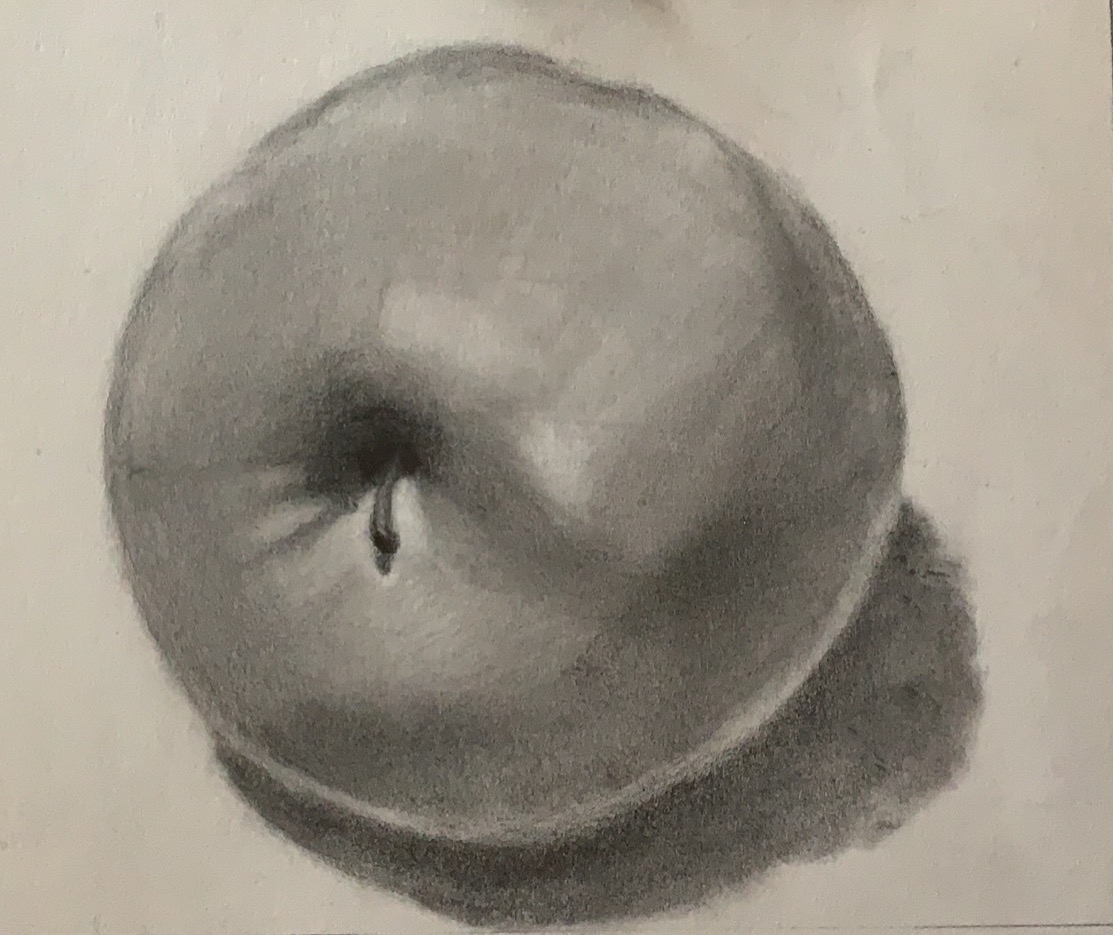A detailed and polished descriptive caption of the given voice-provided information could be:

"This is a meticulously crafted charcoal drawing on a white sketching paper, capturing the intricate details of an apple. Rendered in grayscale, the apple rests on its side, with its distinct black stem prominently jutting out from the left side. The lighting in the drawing appears to strike from the upper area, casting nuanced shadows that enhance the apple's form and create a defined shadow extending to the right below it. Although the image is predominantly grayscale, a subtle warm hue is noticeable, suggesting that the photograph of the artwork was taken under warm lighting conditions, adding a soft and inviting quality to the composition."